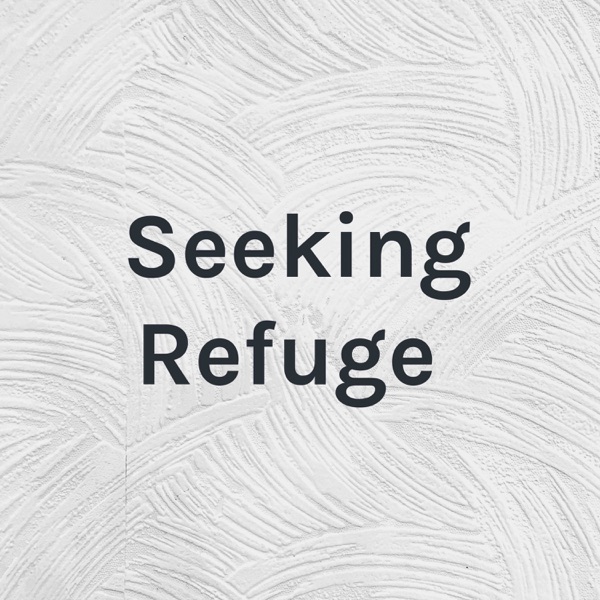The image features a textured white background, covered with ridges and swirling arcs, as if an object or brush was used to create a complex, layered surface. The background includes subtle blue hues and faint swirling patterns that resemble hair. Central to the image are the black words "Seeking Refuge," with the word "Seeking" capitalized and positioned above the word "Refuge." Notably, the "G" in "Refuge" has a distinctive, ornamental curly shape. The background, which suggests multiple layers of paintwork, includes a vertical seam that starts in the lower left corner and extends to the upper left corner, resembling sections of drywall painted over. This seam is the only prominent feature apart from the textured surface and the central black text.